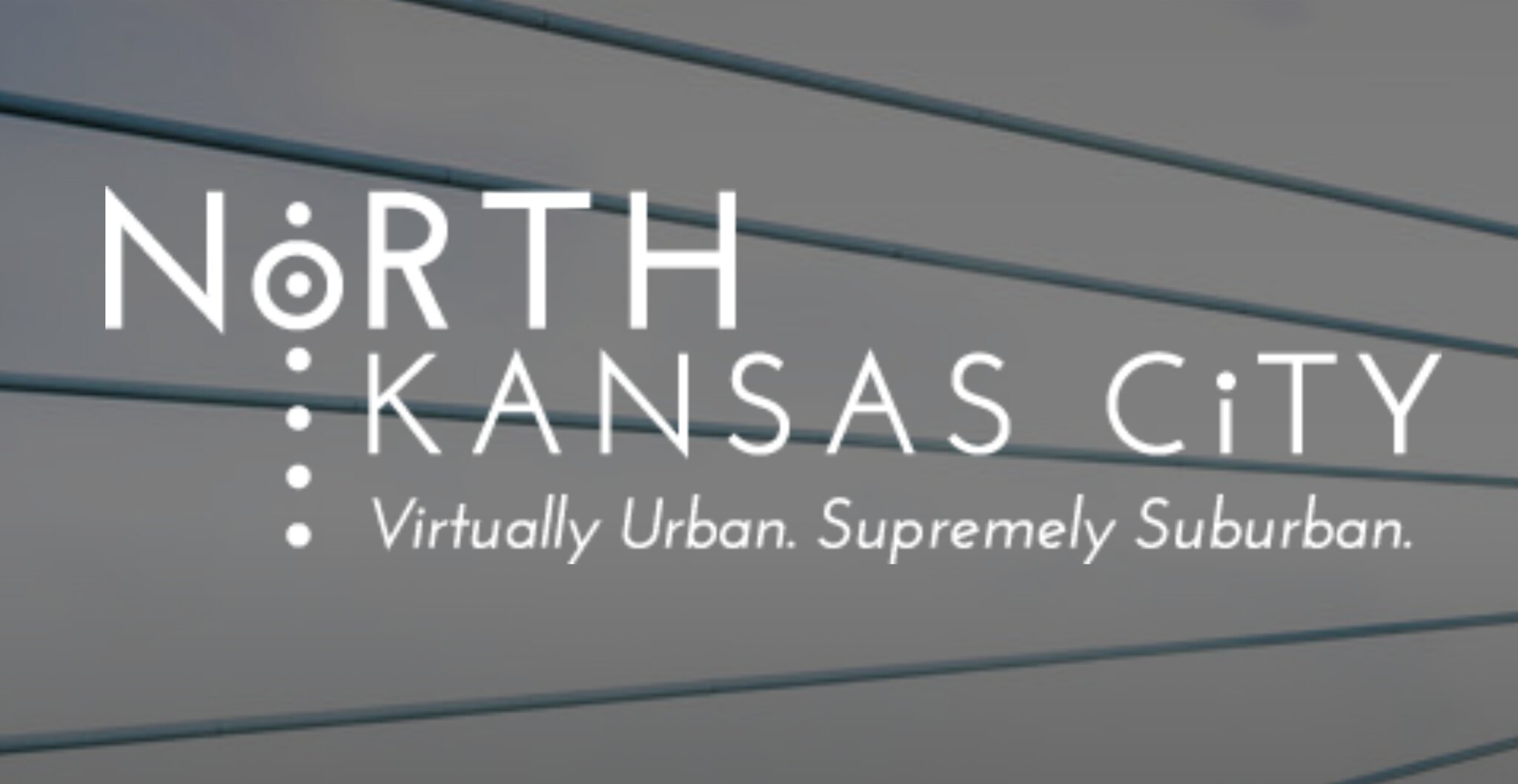The image features a gray, sloped, siding-like background with bold, white text that reads “North Kansas City.” The word "North" is distinctive, with its letters larger, and its "O" containing a white dot surrounded vertically by four additional dots, creating a striking visual sequence. Just underneath, "Kansas City" is written in uniform white lettering. Below this, in smaller italicized white font, is the slogan “Virtually urban, supremely suburban.” The background consists of dark, angled lines that may suggest either the seams of a wall or four posts, enhancing the overall sparse and clean design of the advertisement.